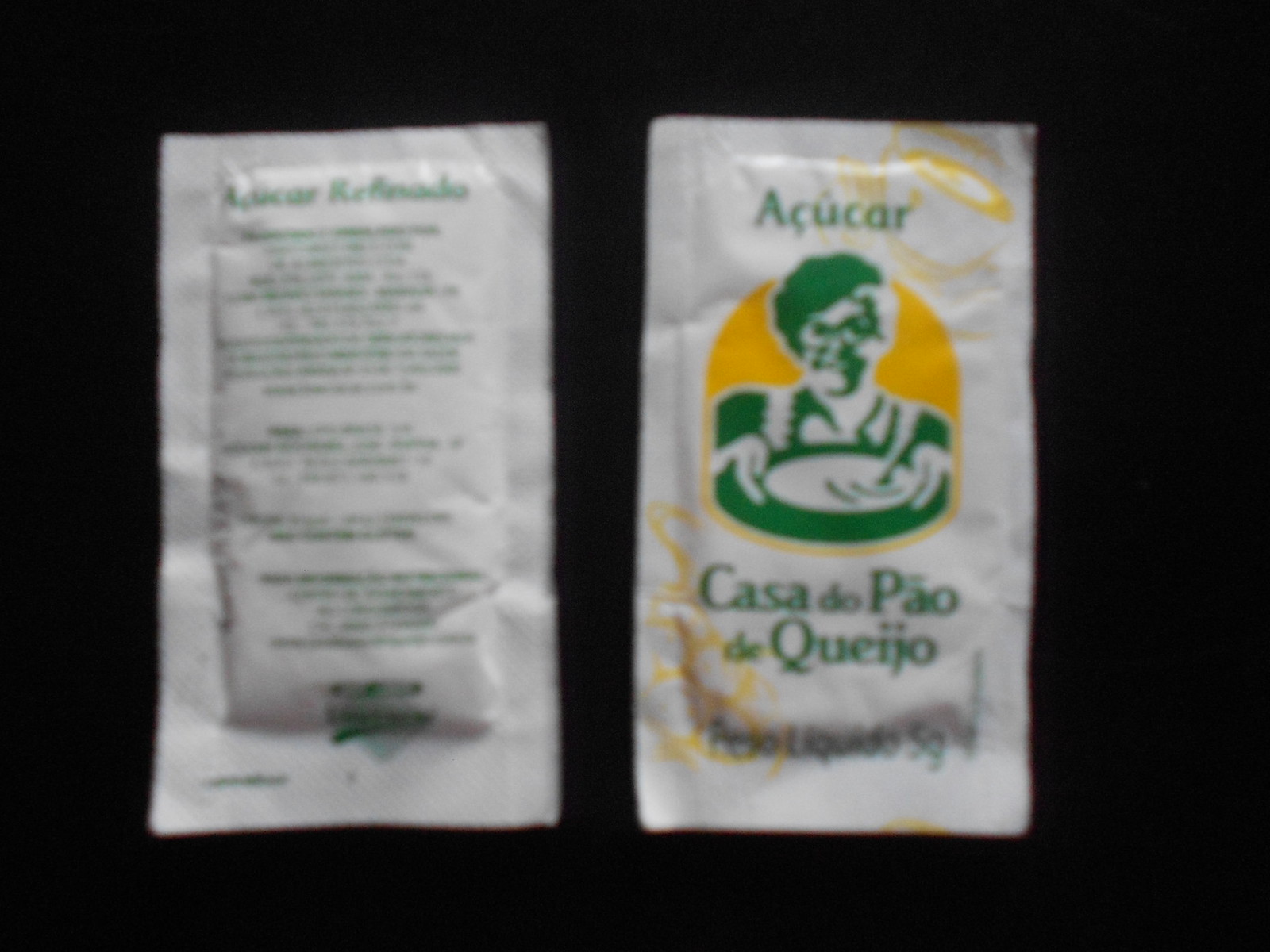The image depicts two small packets, likely containing a Mexican condiment or seasoning. One packet shows the front design, featuring a white background with green lettering and a yellow background behind a smiling Hispanic woman with short hair and glasses. She is wearing a dress and an apron while holding a bowl, which some describe as containing soup. The text on the front reads "Acucar" and includes the phrase "Casa de Peo de Cujillo," along with additional text that is unreadable. The second packet shows the back side with several lines of text, presumably the ingredients, which are hard to make out. Both packets are placed against a dark gray or nearly black surface, possibly a table or wall.